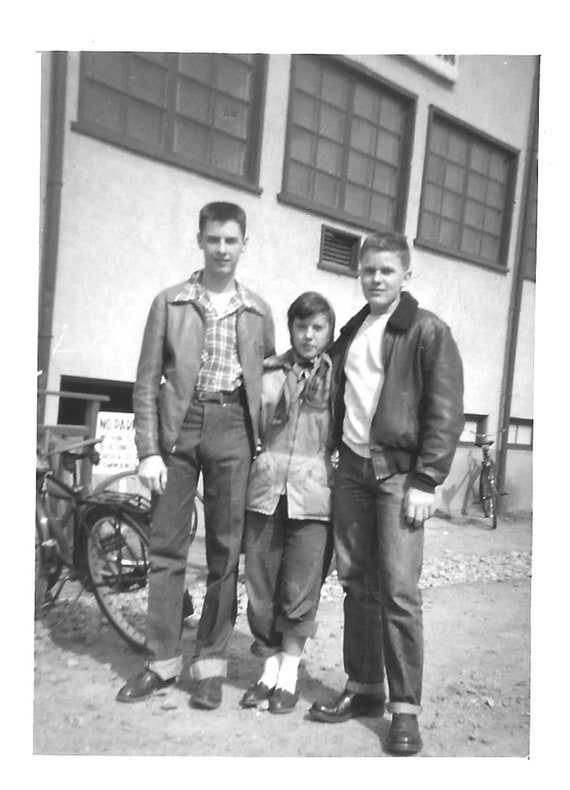This detailed black-and-white photograph, likely from the 1950s or early 1960s, captures three young people—two boys and a girl—standing in front of what appears to be a school building. The ground beneath them is an unpaved, rocky dirt road, with a light gray hue. A row of light gray stones lines the foreground, adding texture to the scene.

In the left corner, there is a dark-colored bicycle leaning against a dark fence, contributing to the vintage atmosphere. Behind this fencing, we see squat, black-framed rectangular windows, one of which has a distant second bicycle resting against the wall. Higher up on the wall, three large, gray-rimmed windows with numerous small panes are visible, each contributing to the building's old-timey charm. A ventilation vent is situated under the middle window.

The trio stands in the center of the frame. On the left is a tall boy with a dark, buzz-cut hairstyle. He is dressed in blue jeans with rolled-up hems, dark pointed shiny shoes, and a mid-gray leather jacket over a tucked-in collared, checkered shirt. His left arm is affectionately around the girl in the middle.

The girl in the center, who is shorter than the boys, wears dark pants rolled up almost to the knees, white socks paired with black shoes, and a headscarf tied around her head, adding a touch of modesty and style.

To the right, the second boy wears dark jeans rolled up above the ankles, black shiny shoes, and a thick bomber jacket over a white untucked t-shirt. His hairstyle is a light-colored, slightly taller buzz cut.

All three kids, appearing to be teenagers, stand close together on the dirt road, embodying a snapshot from a bygone era.